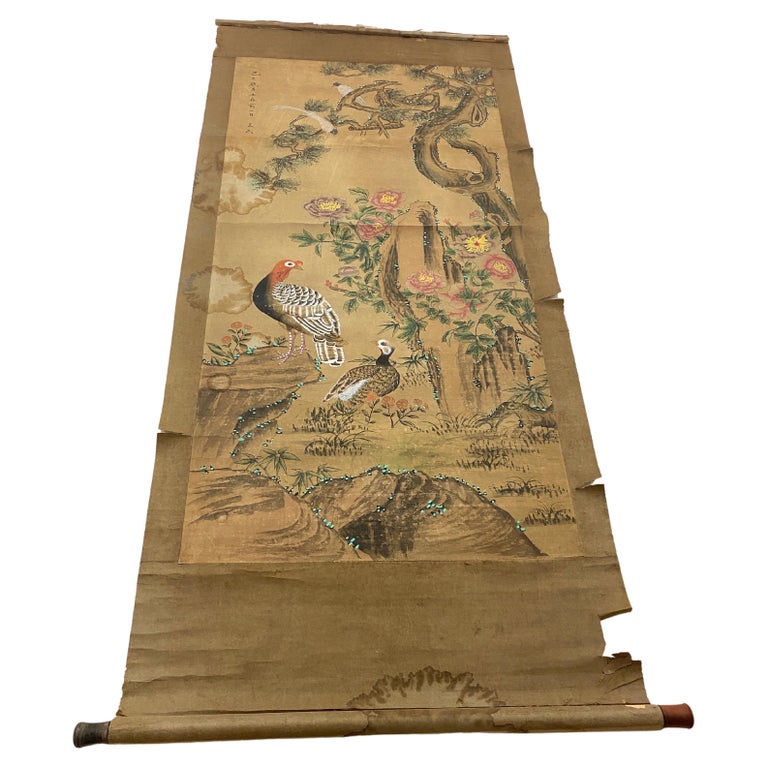This photograph features an unrolled, aged oriental scroll with evident damage, including rips along the sides and water-stained edges, suggesting significant wear over time. The scroll is a dark brown fabric with wooden posts at its ends, allowing it to be rolled up. The intricately detailed artwork depicted within the scroll showcases a tranquil nature scene, dominated by what appear to be peacocks or other large, colorful birds with distinctive red faces and multicolored feathers. The birds are set amid a lush environment featuring vibrant blossoms in hues of purple, pink, and yellow, situated on curved tree branches adorned with pine needle leaves. In the background, a picturesque mountainous landscape with light blue elements and additional floral and arboreal details completes the serene vista. The composition exudes an aesthetic focus on natural beauty rather than scientific accuracy.